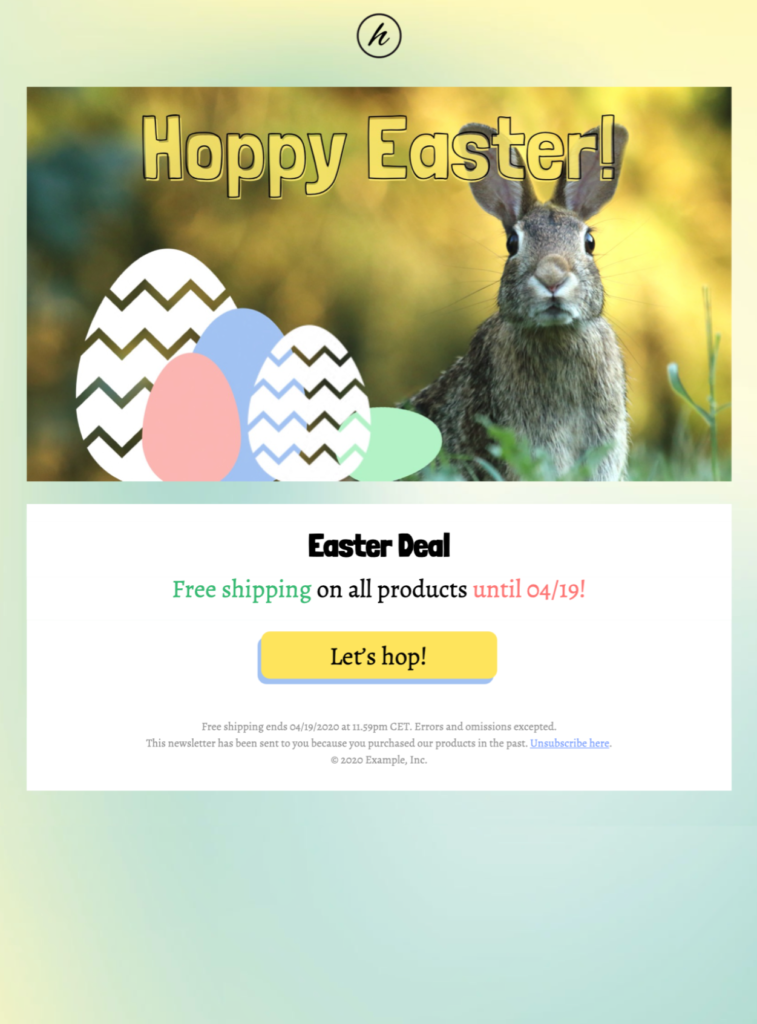This image, likely sourced from a website or email newsletter, features a festive, Easter-themed design. At the top, only a portion of a logo is visible, presenting the letter "H." The central focus of the image is a realistic brownish-gray rabbit sitting amidst digitally created Easter eggs. These eggs come in various colors: white, blue, red, and a smaller green one, with the white eggs having a computer-generated zigzag pattern that mimics cracks. 

The background behind the rabbit is artistically blurred into a yellowish tint, adding depth to the composition. The headline "Happy Easter" is prominently displayed in yellow. Below this, a bold, black text announces an Easter deal offering "Free Shipping on All Products until 04-19!" with the date highlighted in a pinkish-orange hue, and "free shipping" in green, emphasizing the promotional details through varied color usage.

Towards the bottom center of the image, a large yellow button with black text reads "Let's Hop," likely serving as a call-to-action for users. Additional information spans the bottom edge, detailing that the free shipping promotion ends on 04-19 at 11:59 PM and includes an advisory about errors and omissions. The footer of this image mentions that it was sent as a newsletter due to the recipient's past purchases, offering an unsubscribe option and listing a sample year, "2020."

The design rounded off with green hues at the bottom, lends a cohesive and vibrant touch, making it suitable for use as a digital poster or as part of an Easter-themed email. The exact branding remains unclear, indicated only by an "H" logo at the top, which could represent a company name or initial.